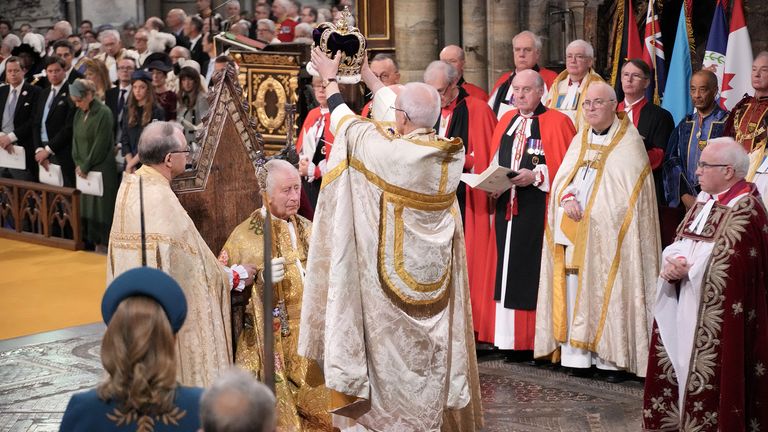This detailed photograph captures the coronation ceremony of King Charles in England. King Charles, clad in an opulent gold robe with white gloves, sits on a rough, wooden throne. He holds a staff matching the color of his robe. Before him stands a man in a beige and gold robe, holding a black and gold crown with white trim aloft in both hands, preparing to place it on King Charles' head. Surrounding them, a diverse crowd of attendees is donned in an array of ceremonial attire, including red cloaks, white and black robes, and gold-decorated garments. Notably, a woman in the foreground sports a green hat and matching suit coat, her brown hair curled at the ends. Behind her, a balding man and other spectators observe the scene. The setting is a historic building with gray stone floors and stone pillars in the background, contributing to the solemn atmosphere. Flags and other regal decorations underscore the significance of the moment, marking the transformation of Prince Charles into King Charles.